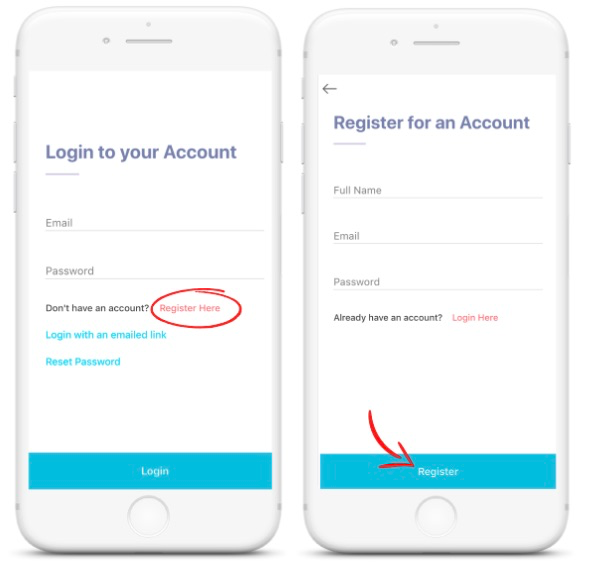The image consists of two screenshots of a white cell phone displaying different stages of a user account interface. 

The first screenshot shows the login page. At the top, there is a prompt that reads "Log into your account." Below this prompt, there are two text input fields labeled "Email" and "Password." Beneath these fields is a message that states, "Don’t have an account? Register here," with "Register here" highlighted in red and circled by a red oval. Further down, there are two blue hyperlinks: "Log in with an email link" and "Reset password." At the bottom of this screen is a grey button labeled "Log In."

The second screenshot depicts the registration page. The top of this page displays the instruction, "Register for an account." Below are fields for users to input their "Full Name," "Email," and "Password." Under these fields, there is text that reads, "Already have an account? Log in here," directing users back to the login page. At the bottom of this screenshot, there is a large blue button labeled "Register," which is accentuated by a red arrow pointing towards it.

These screenshots likely serve as visual instructions for users on how to register for a new account and log in to an existing one.